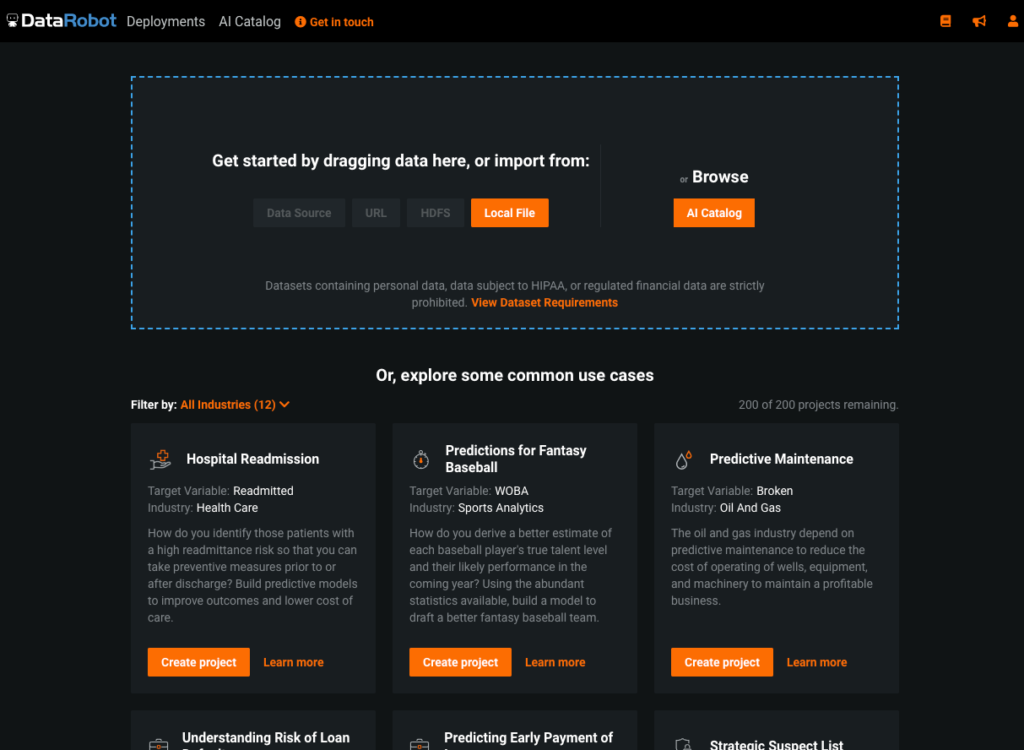A screenshot is displayed, showing a computer screen with a black background. Central to the image are rectangular sections outlined, designed for user interaction and data management. At the top, a prominent, elongated rectangle bordered in blue dots features a prompt that reads, "Get started by dragging data here or import from." This suggests a data import interface on the DataRobot Deployments platform. 

To the right, elements are highlighted in yellow, including the user account information and two unspecified tools, which are available for selection but their functions remain unclear. 

Towards the bottom of the screen, square boxes are visible, each representing different projects. Examples of the projects include "Hospital Readmission," "Predictions for Fantasy Baseball," and "Predictive Maintenance." These areas seem designated for data project management or creation.

At the top of the interface, there is a section labeled "AI Catalog" and a noticeable call-to-action button in orange-yellow stating "Get in touch." The overall layout suggests a user-friendly interface for managing and creating predictive analytics projects.